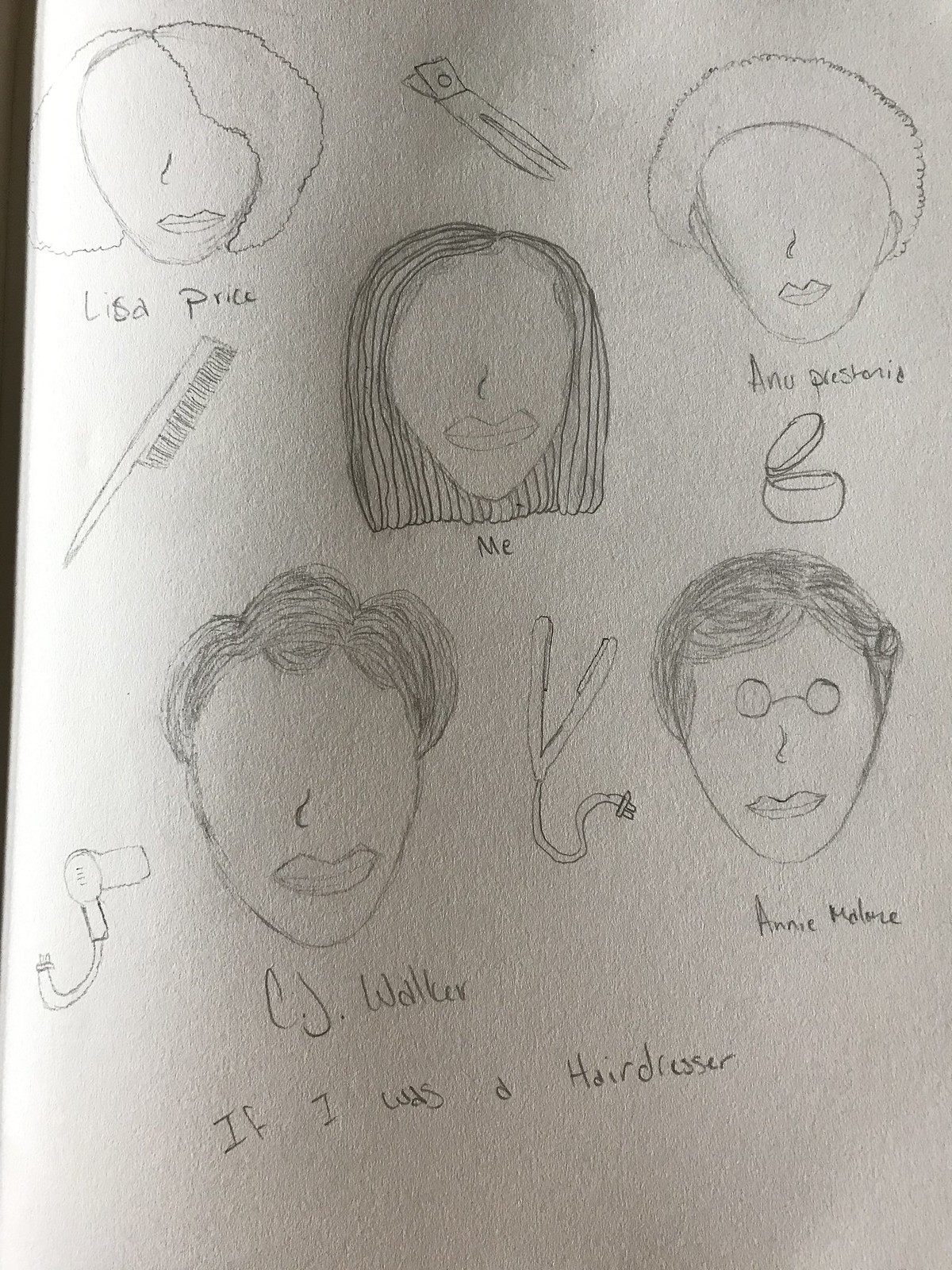A detailed pencil sketch on a white piece of paper, titled "If I Was a Hairdresser," features five faces with distinct hairstyles, noses, and mouths, but notably without eyes. The only exception is the figure in the bottom right, who wears glasses, but no eyes are visible behind them. Below each face, names are labeled: Lisa Price (top left, with bobbed hair and an adjacent pair of unknown hairdressing tools), A New Prestonia (top right, characterized by Afro-esque hair and what appears to be a blush bottle), "Me" (center, with shoulder-length hair and a nearby comb), C.J. Walker (bottom left, with wavy hair and a blow-dryer), and Annie Malone (bottom right, with short hair and glasses, accompanied by a straightener). Tools such as a comb, hairdryer, straightener, and possibly scissors or a blush bottle are placed near the respective faces, enhancing the hairdressing theme.